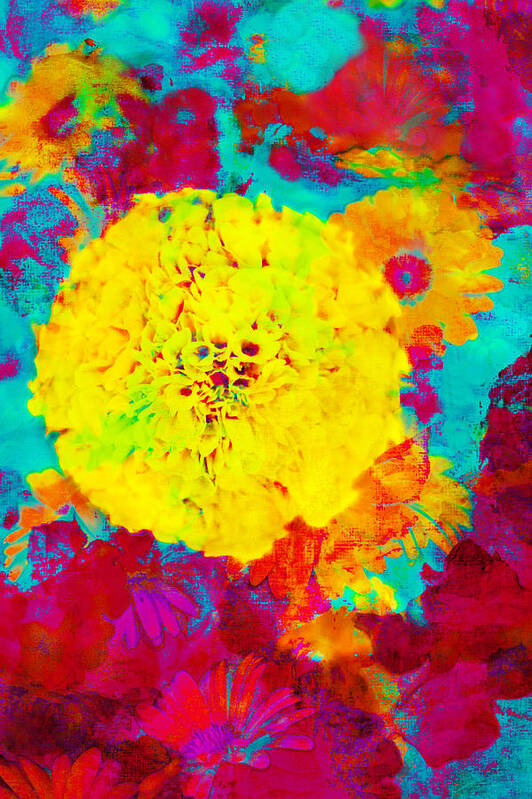This abstract painting features a striking and surreal floral composition, dominated by a large, round, bright yellow flower resembling a marigold or carnation at its center. The densely packed petals of this flower are interspersed with shades and dots of red and green. Radiating out from this focal point are various smaller and more abstractly rendered flowers and petals in vibrant hues. 

To the right of the central flower, another yellow flower with longer, more spaced-out petals and a red center can be seen. The upper left of the painting showcases an orange flower amidst splashes of reddish and purplish hues. Similarly vivid red, purple, and pink splotches appear in the upper right and lower left corners, contributing to the dynamic color scheme.

The entire composition is set against a vibrant teal blue background, accented with turquoise and interspersed with floral imagery, enhancing the painting's surreal and visually striking effect.